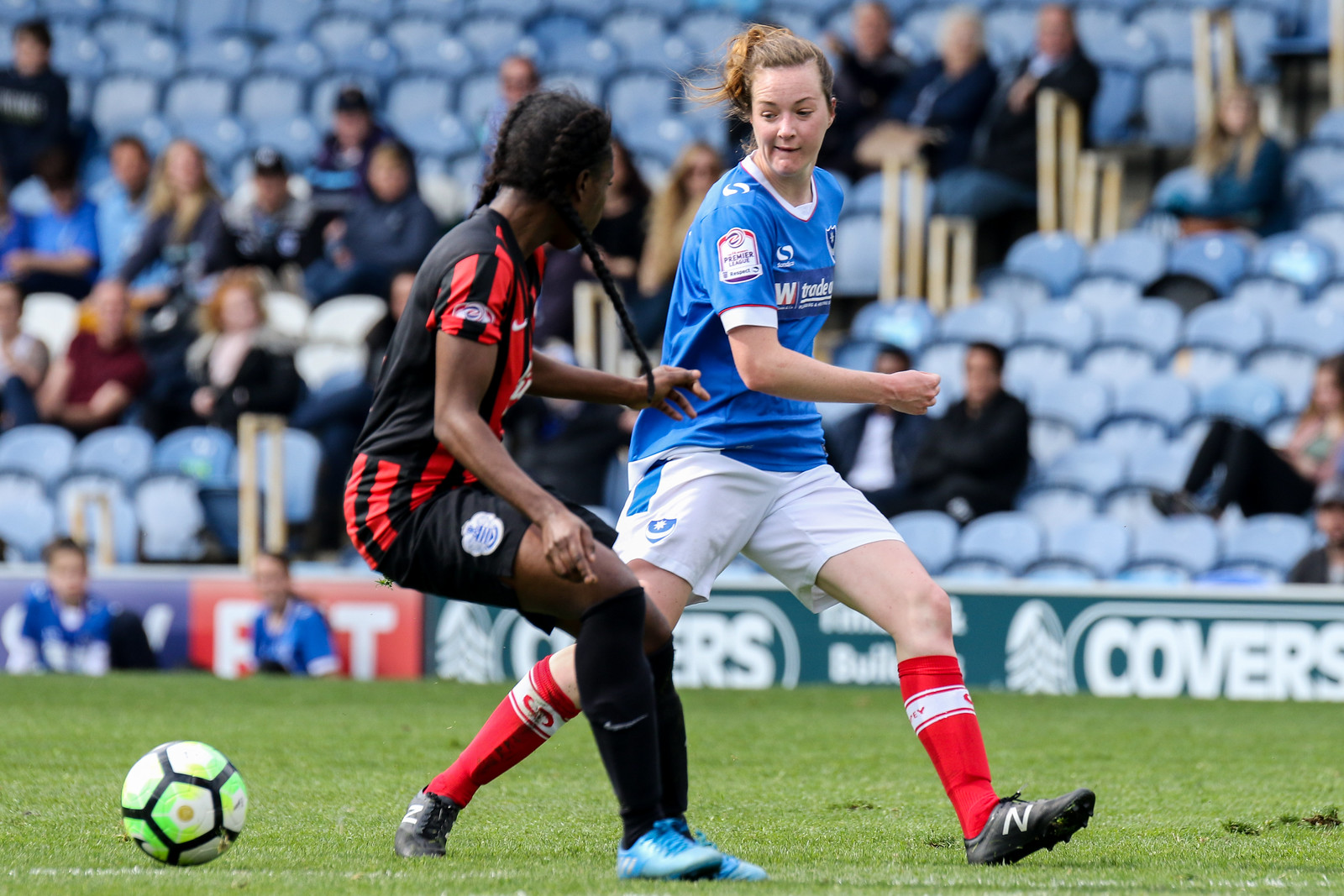The image captures an intense moment in a soccer match featuring two teenage female players in action. The player on the left, an African-American girl, wears a black jersey with red vertical stripes, black shorts, long black Nike socks, and blue shoes. Her opponent, a white girl with brown hair, dons a blue jersey, white shorts, long red socks, and black New Balance cleats with the letter 'N' prominently displayed. Both players appear focused and intense as they play, with the soccer ball positioned on the green grass field behind them. The ball is noticeably green, white, and black. The backdrop features a partially filled stand with white seats adorned with blue tops, and a somewhat blurry wall bearing the word "COVERS" in large white letters against a blue background. The scene suggests a live match with an active audience watching the unfolding drama on the field.